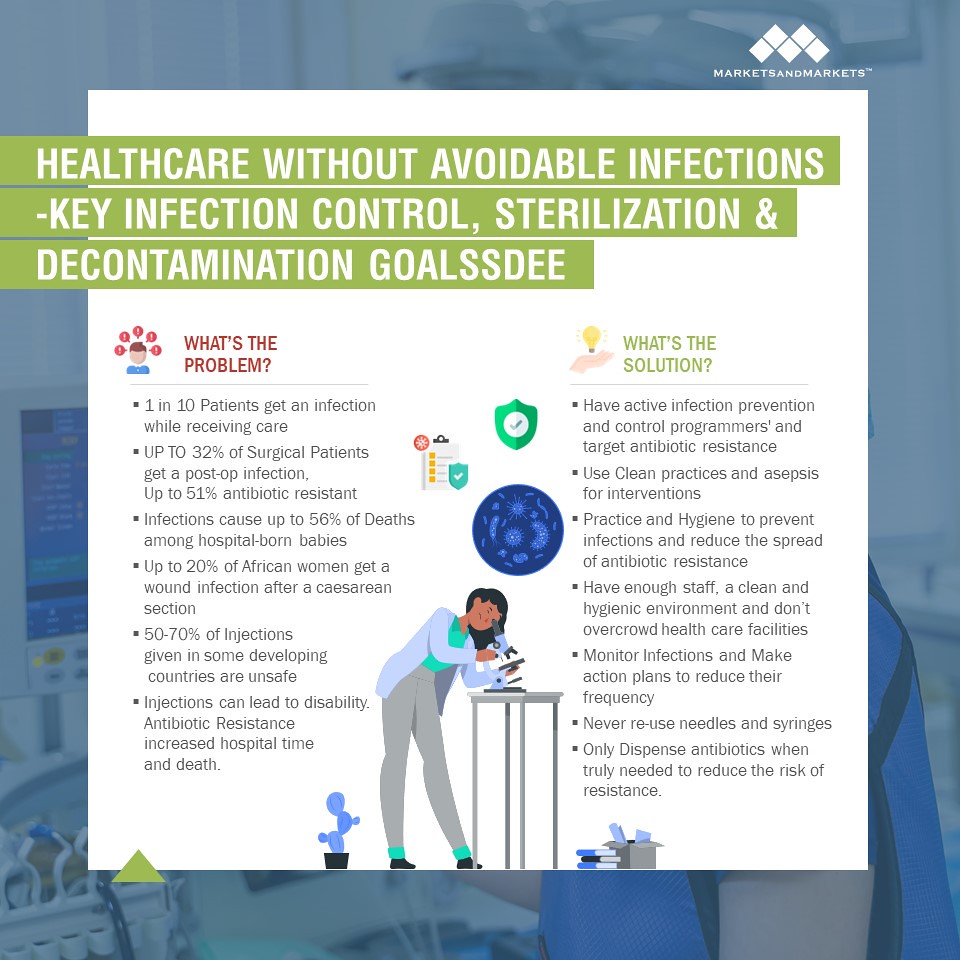The infographic provides valuable information on preventing healthcare-associated infections. It features a blue border with a partially obscured image of a medical operation in the background. Dominating the center is a white box containing essential details, overlaid with a green banner that reads, "Healthcare without avoidable infections: key infection control, sterilization, and decontamination goals." 

The infographic is divided into two main sections. On the left, under the red header "What's the problem?" it details alarming statistics: 
- 1 in 10 patients gets an infection while receiving care.
- Up to 32% of surgical patients get post-op infections.
- Up to 51% of infections are antibiotic-resistant.
- Infections cause up to 56% of deaths among hospital-born babies.
- Up to 20% of African women get wound infections after caesarean sections.
- 50-70% of injections in some developing countries are unsafe, leading to disabilities, antibiotic resistance, extended hospital stays, and death.

An image on this side shows a female scientist looking into a microscope while other illustrations depict germs, a checklist, and a green shield with a checkmark.

On the right, titled "What's the solution?" it lists measures to combat these issues:
- Implement active infection prevention and control programs.
- Target antibiotic resistance.
- Use clean practices and asepsis during interventions.
- Practice good hygiene to prevent infections and reduce antibiotic resistance spread.
- Maintain adequate staffing and a clean, hygienic environment; avoid overcrowding healthcare facilities.
- Monitor infections and develop action plans to reduce their frequency.
- Never reuse needles and syringes.
- Dispense antibiotics only when truly needed.

In the top right corner, the infographic is credited to "Markets and Demarkets."

This comprehensive resource aims to educate the public on the importance of infection control and the necessary steps to prevent healthcare-associated infections.